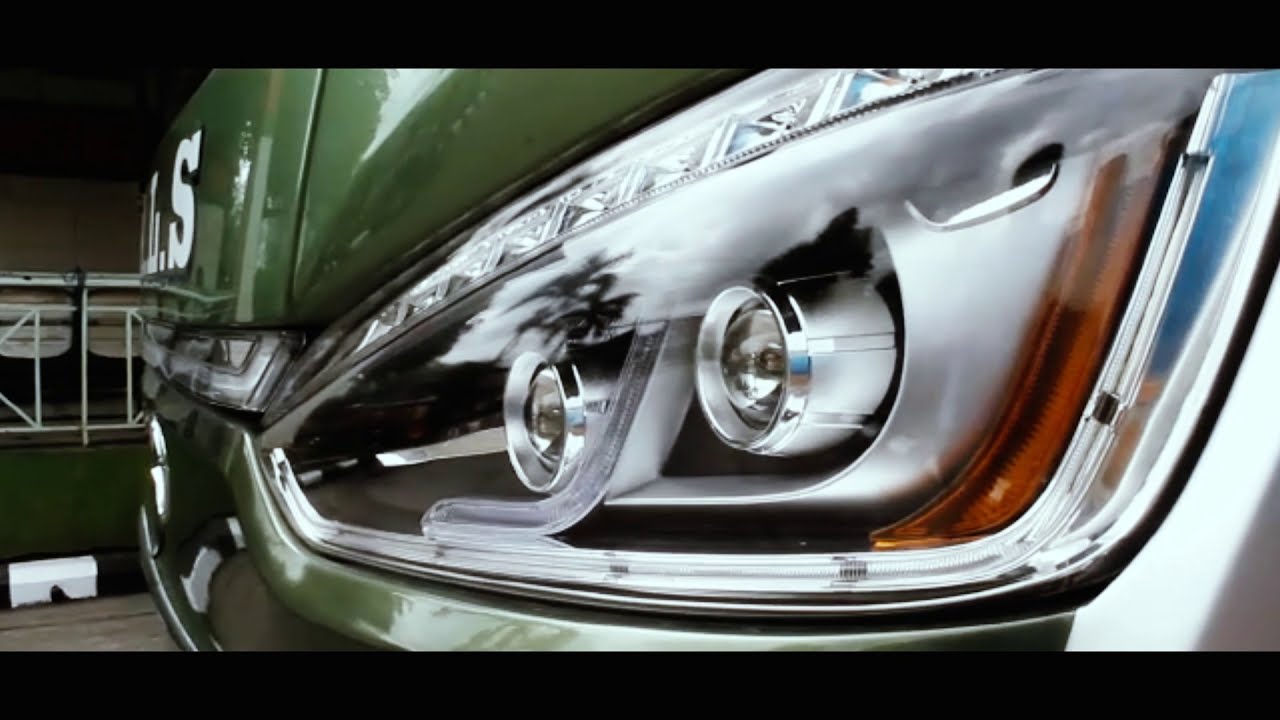The image depicts a very close-up view of the headlight assembly on the left side of a green vehicle, possibly a car or truck. The headlight features two circular bulbs, and to the left of these is a vertical band of orange, presumably a turn signal light. The vehicle's body is a dark, perhaps forest or army green. The bumper is chrome, and there is some lettering on the front of the vehicle; only an "S" is discernible, as the rest fades into the background. Surrounding the headlight is a distinctive plastic casing with a design extending from left to right. The background includes a green cement wall and railing, with a portion of the concrete flooring visible at the bottom left. The image is bordered by black margins at the top and bottom, but not on the sides. Overall, everything appears neat and clean.